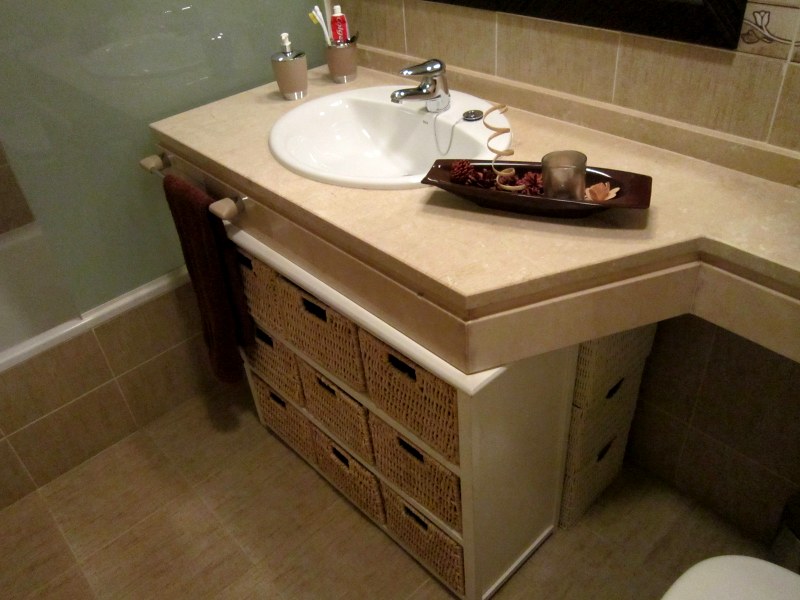This image showcases a stylish corner bathroom unit in a fawn color, featuring a washbasin that starkly contrasts with its pristine white surface and is equipped with a chromium tap, complete with a chain and plug. Above the sink, the splashback comprises fawnish-greenish tiles leading up to a mirror. A white decorative trim runs along the front of the unit, which appears to have a woven texture resembling sisal or rattan, often seen in small storage units with variously sized drawers.

To the left, there is a white towel rail affixed to the unit, from which a brown towel hangs, adding a touch of warmth to the space. The surface of the unit extends around a corner, narrowing off out of the picture's frame. Atop this work surface sits an oblong dark brown dish, possibly holding potpourri and a candle, contributing to the room's welcoming ambiance. Although the left wall is challenging to discern, it may be part of a surrounding bath area, further adding to the functionality of this thoughtfully designed corner unit.